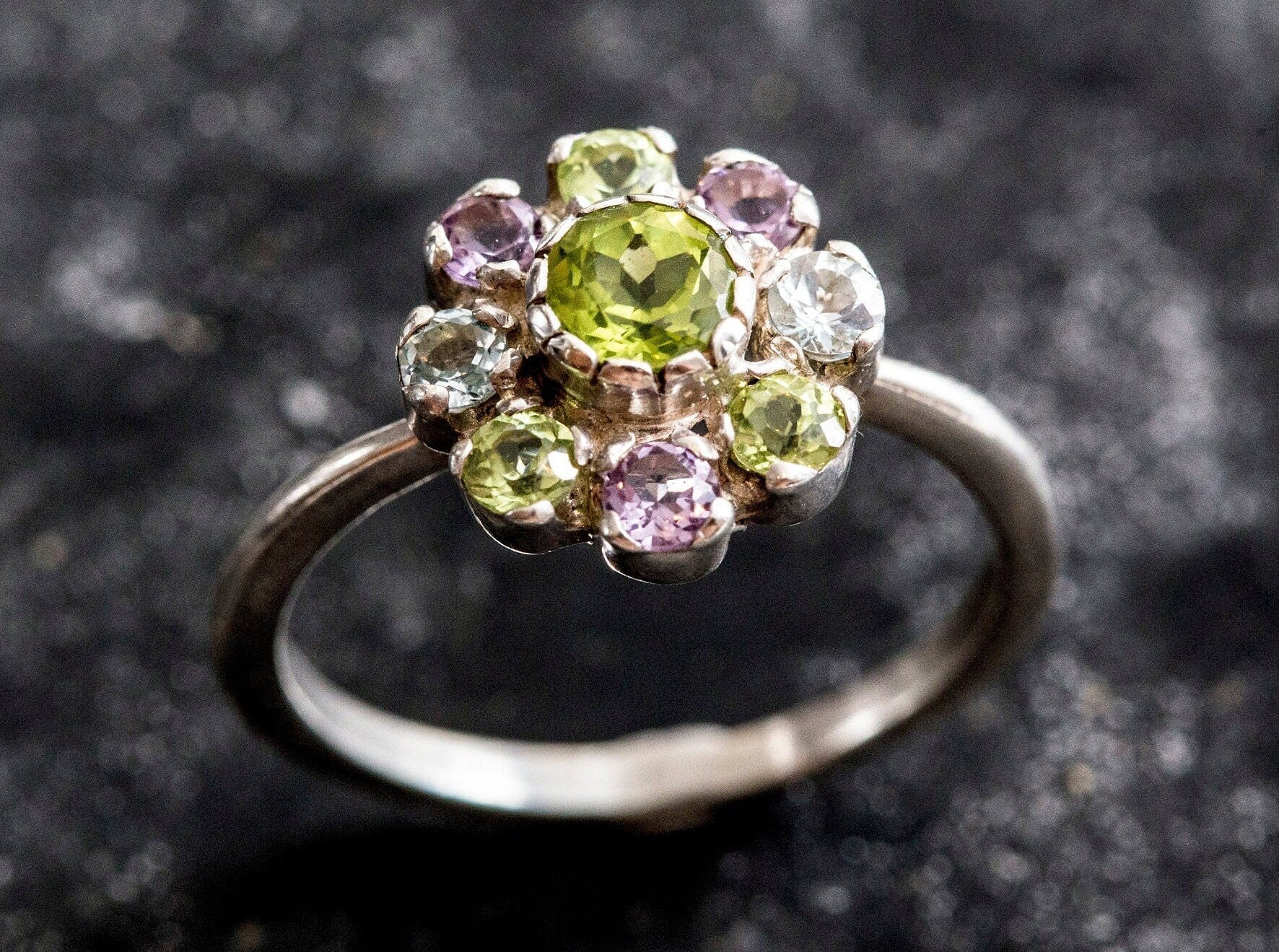This is a highly detailed, professionally taken photograph showcasing a sophisticated ring. The photograph features an up-close view of the ring with impeccable staging, lighting, and focus, set against a blurred, dark background with tones of gray, charcoal, and black speckled with white. The ring itself has a thin, bright silver, possibly platinum or white gold circular band. At the center of the ring sits a large, round yellow gem, which is encircled by a series of eight smaller round gems that form a flower-like arrangement. These surrounding gems consist of various colors, including clear white, light pink, light yellow, and possibly greenish-yellow. There is no text in the image, and all observable colors are accounted for, emphasizing the intricate and vivid details of the jewels.